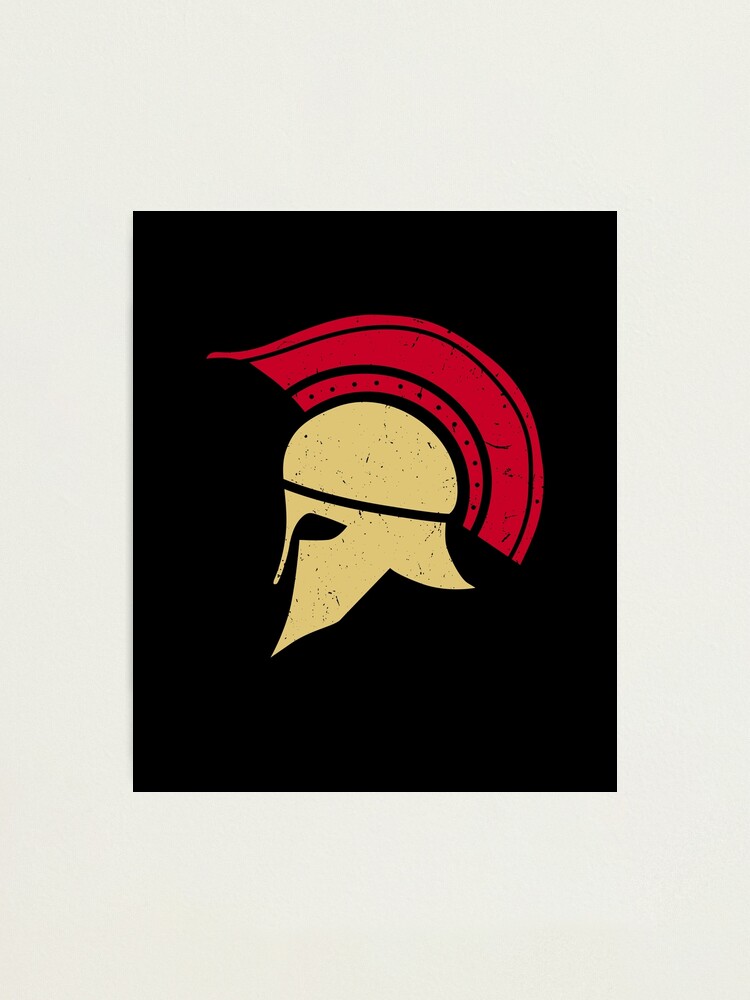This artwork is a minimalistic, rectangular print set against a light gray background. It features a side view of a Spartan or Trojan-style helmet, reminiscent of Roman or ancient warrior helmets similar to those seen in the movie 300. The helmet is predominantly a light gold or cream color with a semi-circular red mohawk running from the front to the back. The helmet, depicted on a solid black background, includes detailed elements such as a pointy nose piece, an eye cutout, and a shield-like ear guard. There's also a black line that resembles a headband blending into the background. The artwork provides textural interest with small black specks on the helmet and mohawk, adding depth to the otherwise smooth surface.